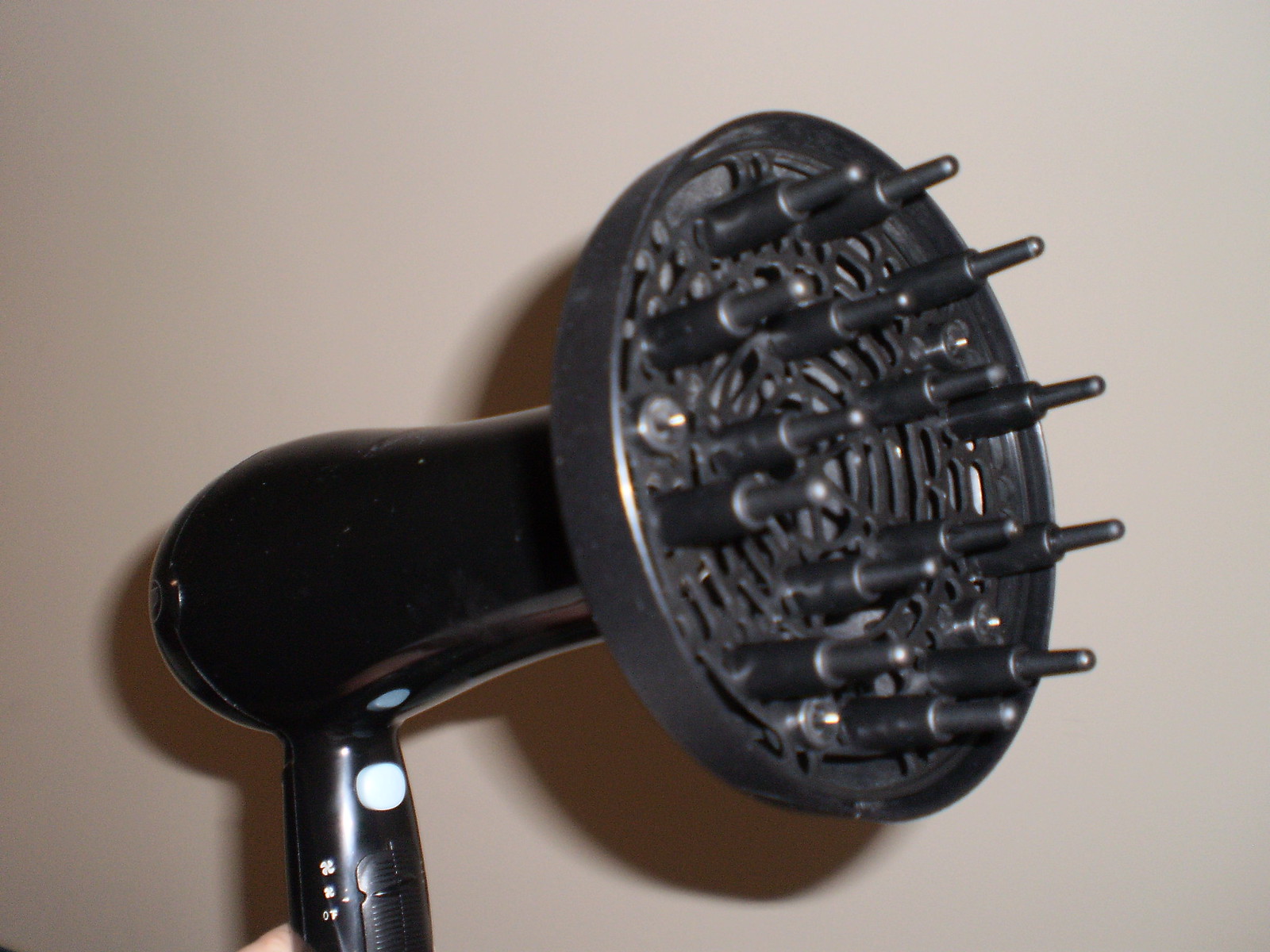This detailed photograph showcases a dark brown, compact hairdryer prominently featuring a large diffuser attachment at its front. Captured against a beige background, the dryer is oriented with the handle emerging from the bottom left corner. The rear of the device is just off the lower left side while the diffuser, occupying the right side of the image, displays an array of prongs and vent openings designed to disperse air. A circular shadow frames the diffuser's head, enhancing its visual prominence. Along the sleek black handle, partially visible settings and a switch for varied heat intensities can be seen. A hand, presumably the left, lightly grips the bottom of the handle, hinting at the manual control of this hair styling tool. This diffuser is particularly effective for individuals with curly or permed hair, aiding in natural drying while adding lift and volume through its pronged design.